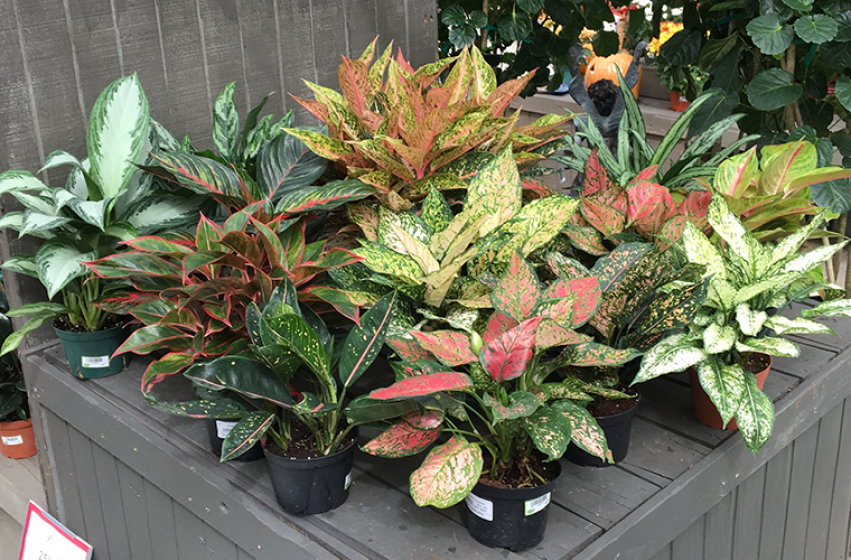This photograph depicts an outdoor setting, likely at a plant nursery or garden center, featuring a large, angled wooden crate made of gray wood, positioned from the bottom left to the top right. Atop the crate rests an abundant array of approximately 20 potted plants, all housed in plastic pots adorned with labels. The plants exhibit a variety of leaf colorations, including solid green, green with red, pink spines, and some with splattered patterns resembling bleach marks. Among them are leaves that are predominantly green with light green or white in the middle, green with yellow speckles, and pink leaves with green speckles. The background reveals additional plants and trees, such as a magnolia tree, along with seasonal decor like a ceramic jack-o’-lantern, suggesting a late summer or early fall timeframe. Additionally, signs are visible in the distance, indicating the commercial nature of the setting.